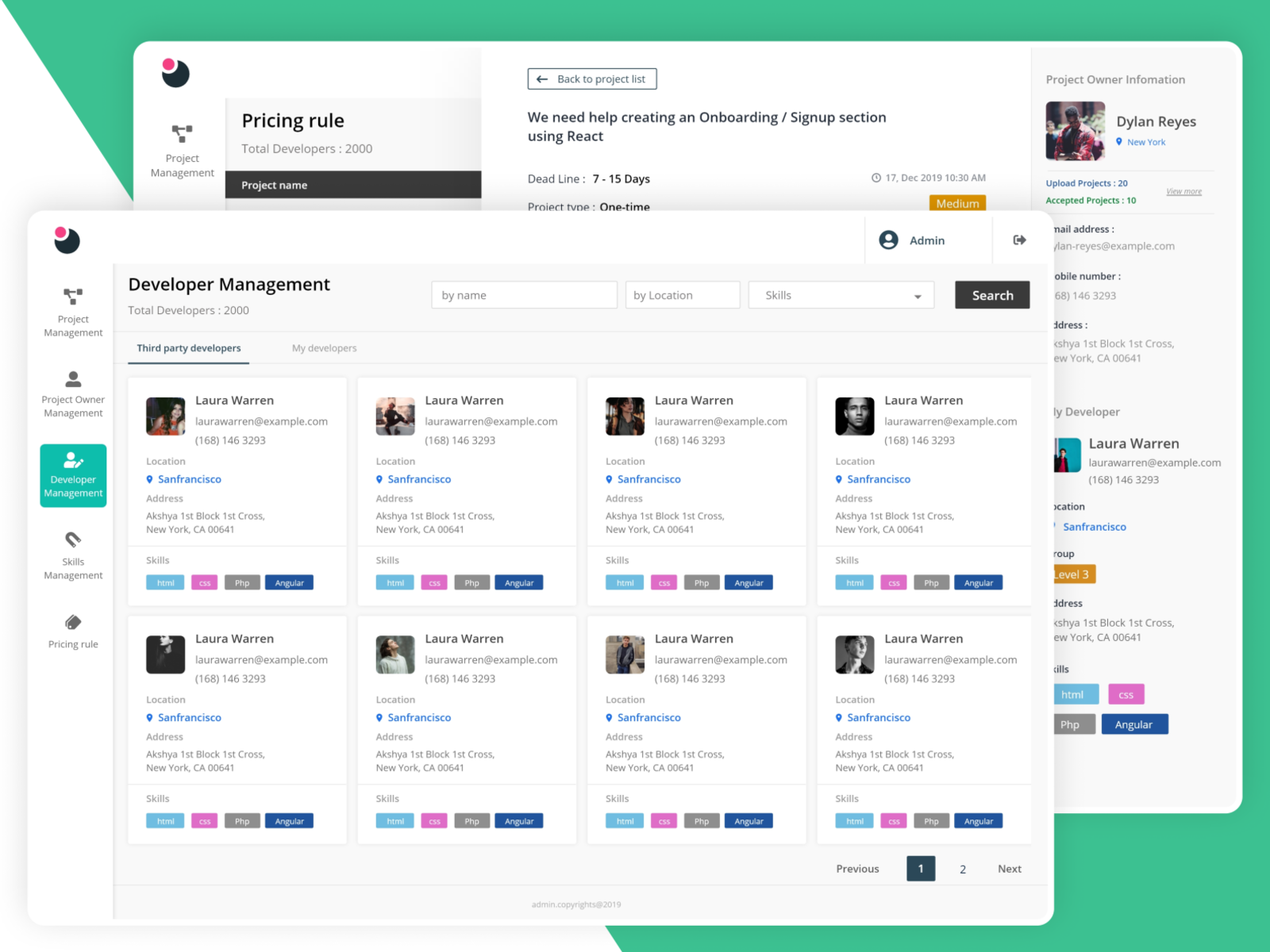The image showcases a detailed project management interface with a green and white background. At the top, it displays a section labeled "Pricing Rule" alongside the total number of developers, which is 2,000. 

On the right side of the interface, within a black rectangle, there's a "Project Name" written in white. Adjacent to that, on the left, there's a "Project Management" tab and a link labeled "Back to Project List."

In the center of the interface, there's a request for assistance in creating an onboarding/sign-up section using React. The project is on a strict deadline, specified to be between 7 to 15 days. Additional project details include: "Product Type: One-time" with a critical delivery date of December 17, 2019, at 10:30 a.m.

The bottom section features an orange rectangle with "Medium" written in white. Accompanying this is a profile picture of a man named Dylan Reeves and his location, "New York," highlighted in blue. Further project information reveals Laura Warren as the project owner.

Moreover, there are three interactive rectangles labeled by name, location, and skills for easier navigation and filtering. A prominent black rectangle contains a search field.

Towards the end, the image depicts a couple of squares featuring profile snippets of different people. The first profile belongs to Laura Warren, and there's indication of a second profile without further details.

This comprehensive layout aims to facilitate effective project management and developer onboarding.